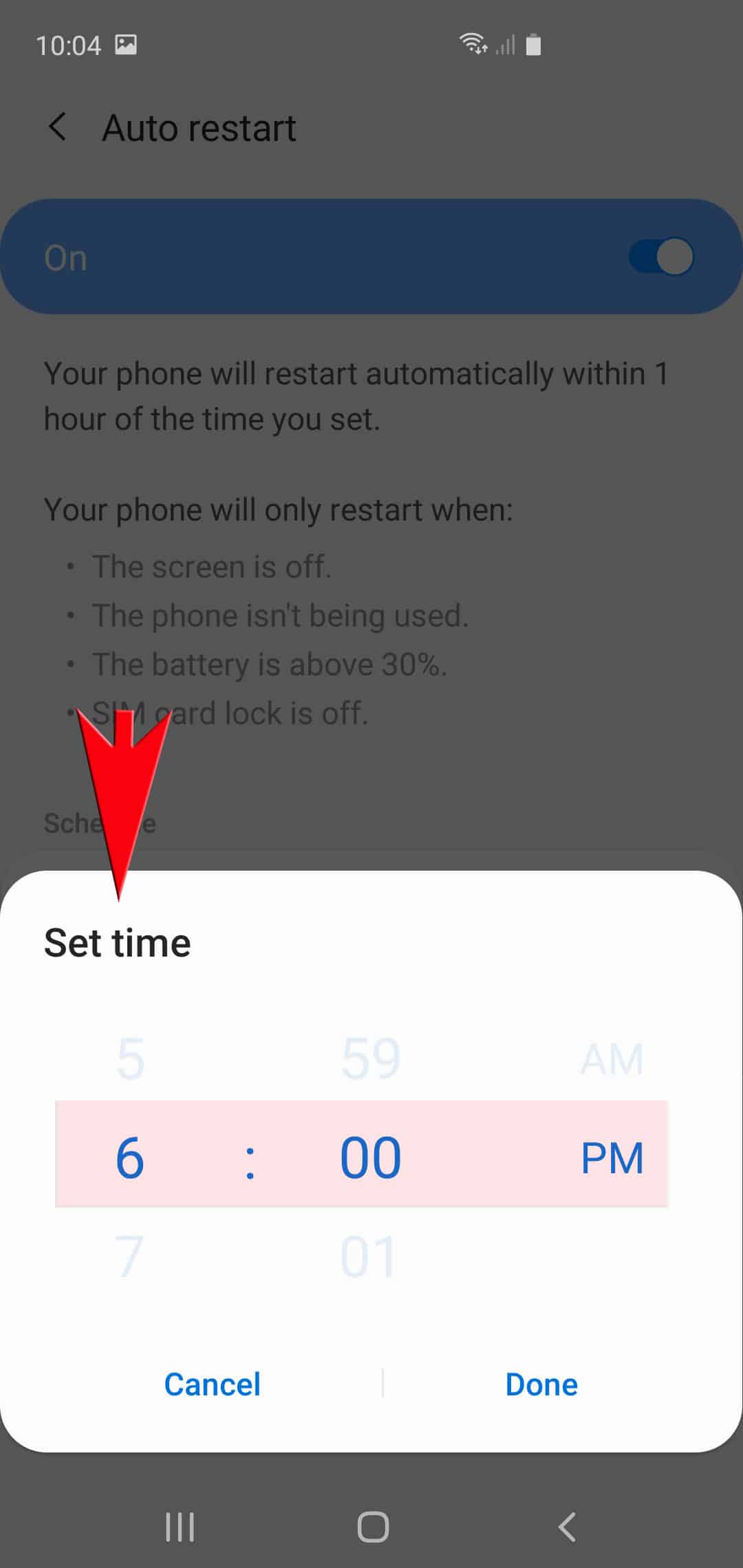The image is a screenshot from an Android mobile device displaying the settings for adjusting the device's time. The main screen is dimmed in the background as a prominent white prompt titled "Set time" occupies the foreground. This prompt features a digital clock interface, allowing the user to scroll through numbers to set the time. The time currently highlighted is 6:00 PM, emphasized in a pink rectangular box. The image includes a red arrowhead pointing down at the "Set time" prompt, clearly added post-capture to draw attention. At the bottom of the prompt, two clickable options, "Cancel" and "Done," are available for confirming or dismissing the action.